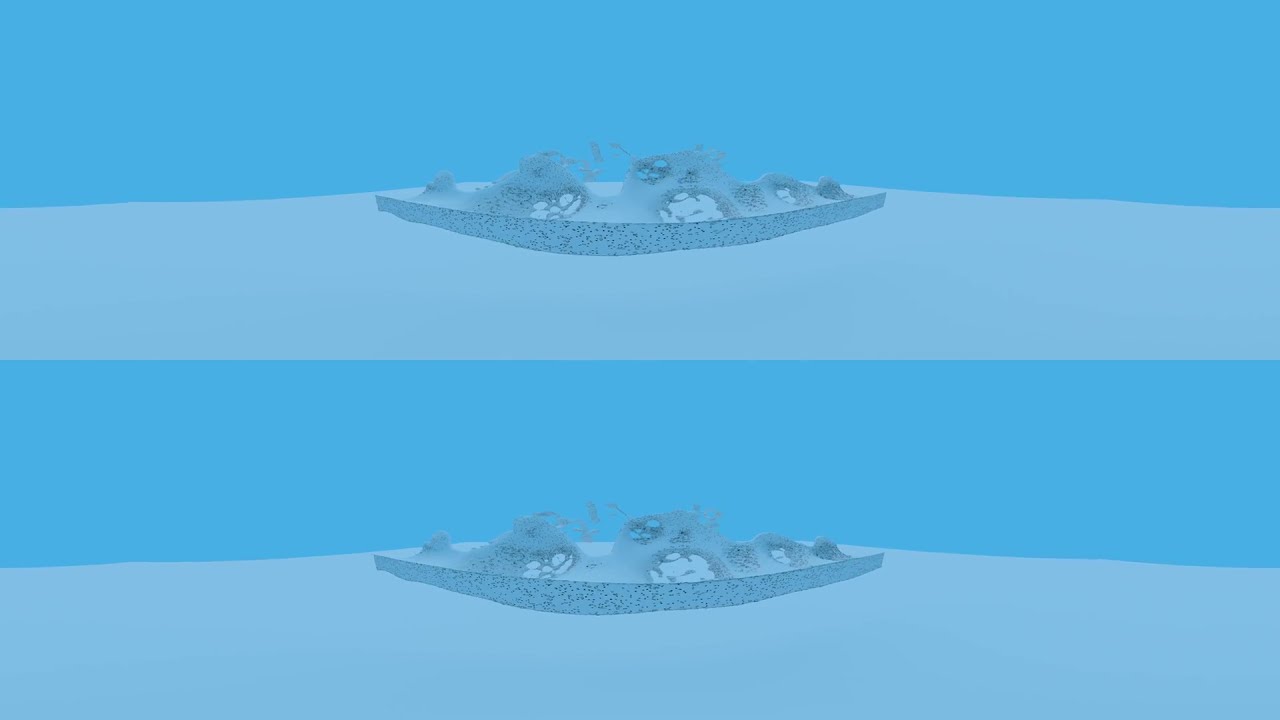The image is a digital or illustrated artwork characterized by its mirrored, repetitive composition. It features a horizontal banner where the same elements are repeated twice. Set against a blue-toned background, the top half showcases a darker blue while the bottom transitions to a lighter blue with a grayish tinge. This lighter blue section curves gently, resembling small hills. In the center of this gradient stands a peculiar structure, mirrored above and below, resembling a semi-collapsed, weathered formation like a broken sandcastle.

This structure is gray and covered with various dark lines and pits, some of which pierce through to the background, suggesting erosion or decay. It possesses a series of four uneven humps and opens in the center and at the sides, adding to its derelict appearance. The bottom sections of the structure blend into darker blue, almost black, mottled areas, further accentuating the weathered, underwater feel. Scattered specks and small attachments protrude from the structure, enhancing its complex, deteriorated aesthetic.